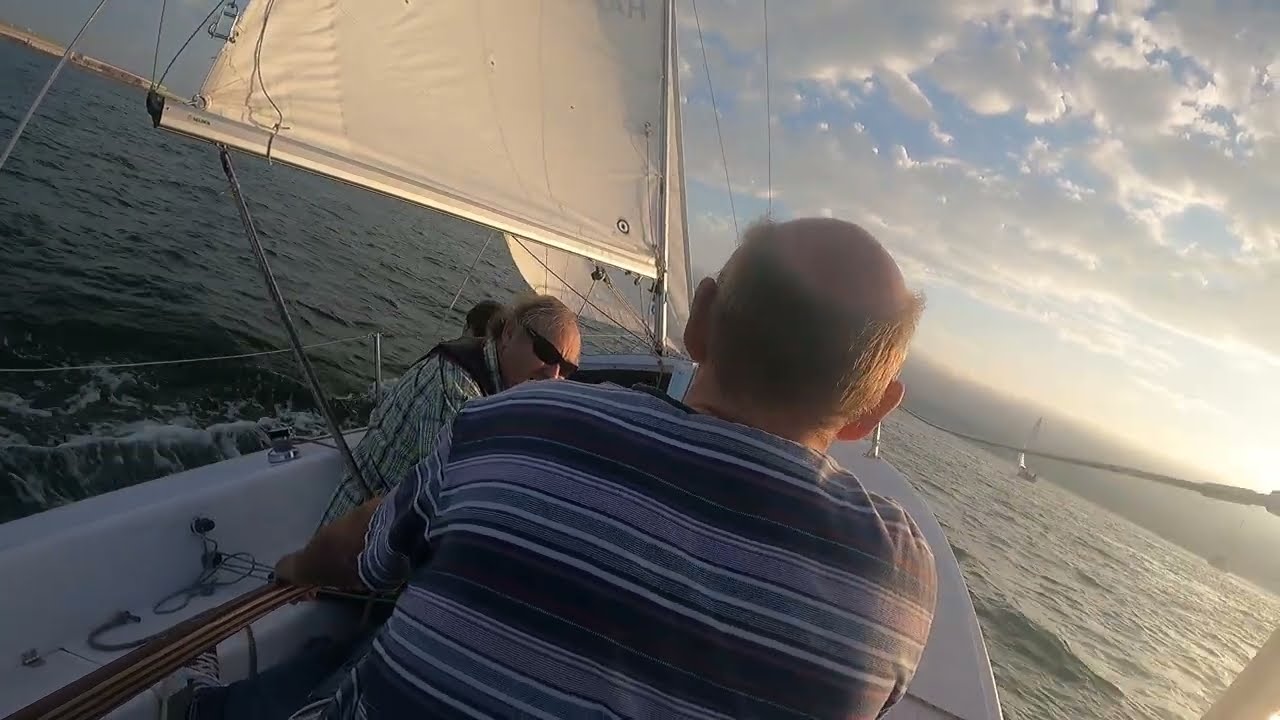In this full-color photograph taken during the late afternoon on a partly cloudy day, we see an outdoor scene of a sailboat on calm waters. In the foreground, two men are positioned on the sailboat. The man closest to the camera, viewed from behind, has light hair and is balding; he's wearing a horizontally striped, short-sleeve shirt. Slightly ahead and to the left of him is another man, also with thinning hair, clad in dark sunglasses and a green plaid shirt. 

The sailboat's white sails are visible on the left side of the frame, catching the wind as the boat turns towards the port side. The water, which is calm but frothing and splashing slightly on the left from the motion of the boat, contributes to the dynamic sense of movement in the scene. In the distance to the right, another sailboat can be seen against the backdrop of the shoreline.

The sky shows patches of blue with fluffy white clouds, and the lighting suggests that the sun is low, possibly indicating an approaching sunset. The overall ambiance of the photograph conveys a serene yet lively sailing experience.